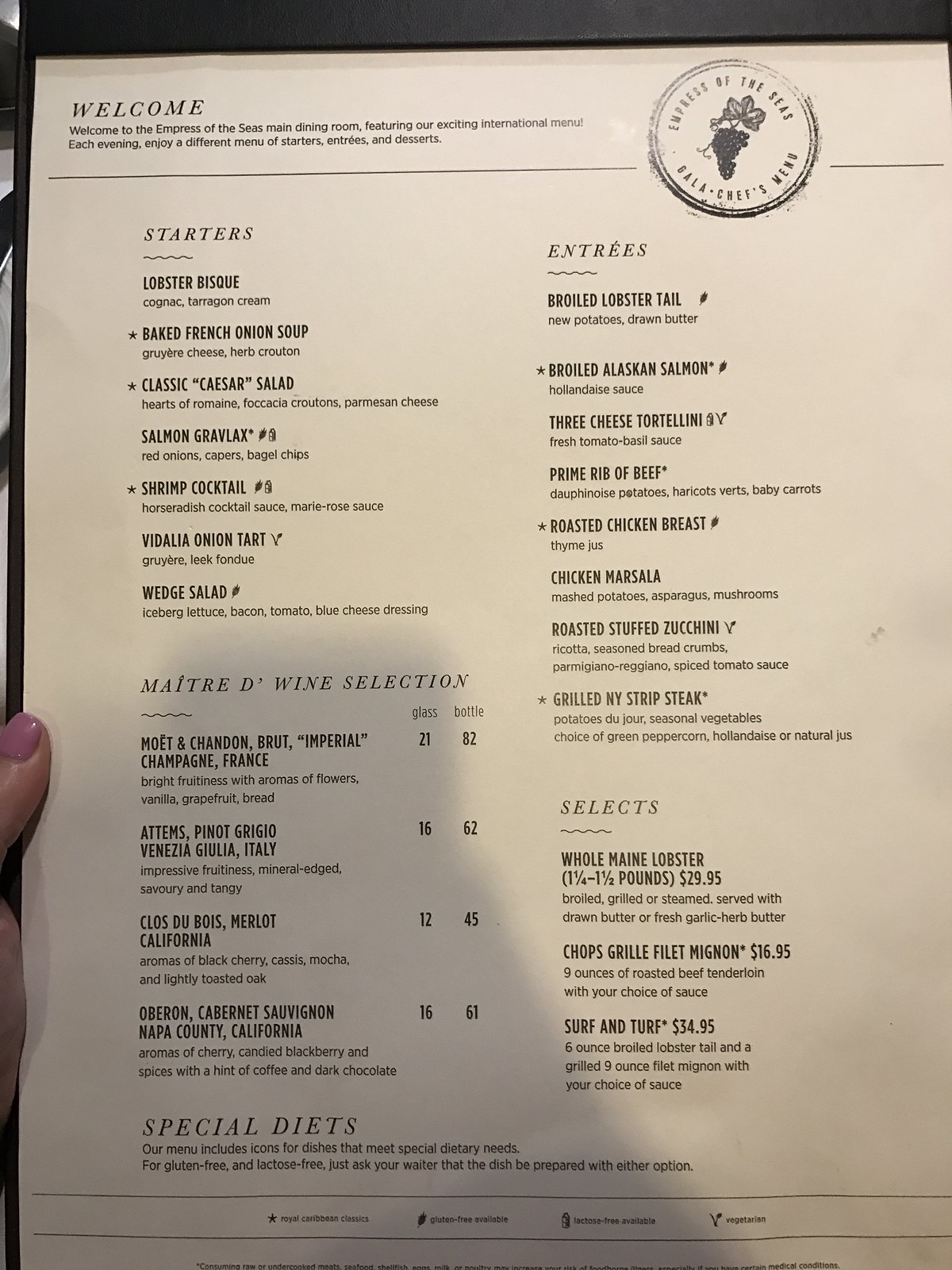**Empress of the Seas Main Dining Room Menu**

**Welcome!**
Welcome to the Empress of the Seas Main Dining Room featuring our exciting international menu! Each evening, delight in a different selection of starters, entrees, and desserts.

**Seal:**
On the right, a seal reads "Empress of the Seas Gala Chef's Menu," with an ornate bunch of grapes at the center.

**Starters:**
- **Lobster Bisque**: Cognac tarragon cream (★)
- **Baked French Onion Soup**: Gruyere cheese herb crouton (★)
- **Classic Caesar Salad**: Hearts of romaine, focaccia croutons, parmesan cheese (★)
- **Salmon Gravlax**: Red onions, capers, bagel chips
- **Shrimp Cocktail**: Horseradish cocktail sauce, Mary Rose sauce
- **Vidalia Onion Tart**: Gruyere leek fondue
- **Wedge Salad**: Iceberg lettuce, bacon, tomato, blue cheese dressing

**Entrees:**
- **Broiled Lobster Tail**: New potatoes, drawn butter
- **Broiled Alaskan Salmon**: Hollandaise sauce
- **Three Cheese Tortellini**: Fresh tomato basil sauce
- **Prime Rib of Beef**: Dauphinoise potatoes, haricots verts, baby carrots
- **Roasted Chicken Breast**: Thyme jus
- **Chicken Marsala**: Mashed potatoes, asparagus, mushrooms
- **Roasted Stuffed Zucchini**: Ricotta, seasoned breadcrumbs, parmigiano-reggiano, spiced tomato sauce
- **Grilled NY Strip Steak**: Potatoes du jour, seasonal vegetables, choice of green peppercorn, hollandaise, or natural jus

**Maitre d' Wine Selection:**
- **Moët & Chandon, Brut Imperial Champagne, France**: Glass $21, Bottle $82. Bright fruitiness with aromas of flowers, vanilla, and grapefruit bread.
- **Attems, Pinot Grigio, Venezia Giulia, Italy**: Glass $16, Bottle $62. Impressive fruitiness, vanilla edge, savory and tangy.
- **Clos du Bois, Merlot, California**: Glass $12, Bottle $45. Aromas of black cherry, cassis, mocha, and lightly toasted oak.
- **Auberon, Cabernet Sauvignon, Napa County, California**: Glass $16, Bottle $61. Aromas of cherry, candied blackberry, spices with a hint of coffee and dark chocolate.

**Selects:**
- **Whole Main Lobster** (1 ¼ to 1 ½ pounds): $29.95. Broiled, grilled, or steamed, served with drawn butter or fresh garlic herb butter.
- **Chops & Grill Filet Mignon**: $16.95. Nine ounces of roasted beef tenderloin with your choice of sauce.
- **Surf and Turf**: $34.95. Six-ounce broiled lobster tail and a grilled nine-ounce filet mignon with your choice of sauce.

**Special Diets:**
Our menu includes icons for dishes that meet special dietary needs. For gluten-free and lactose-free options, please ask your waiter to prepare the dish accordingly.

**Symbol Key:**
- Star (★) denotes Royal Caribbean classics.
- Wheat symbol indicates gluten-free options available.
- Milk carton symbol indicates lactose-free options available.
- V denotes vegetarian options.